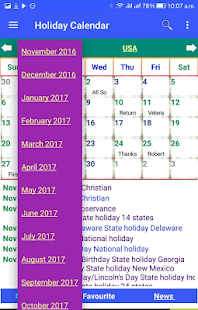This image depicts a detailed holiday calendar displayed on a smartphone screen. The top and bottom bars of the screen are blue, framing the central content. At the very top, a horizontal blue box spans the width of the phone, indicating it is currently 10:07 AM with a battery life of approximately 78% and a strong network connection. The title "Holiday Calendar" is prominently displayed in white text, accompanied by a clickable search bar and a menu icon represented by three vertical dots, indicating that it has been accessed.

The calendar covers a range from November 2016 to October 2017, though it appears to skip certain months. The main calendar content features white date boxes and a green strip at the top labeled "USA." To the right of the calendar is a purple drop-down box with green text indicating the current month, "November." To the left of this purple drop-down, there is a section labeled "Christian" and "Christian observance," likely highlighting specific holidays and their descriptions. The text descriptions alternate between black and blue for better readability.

At the bottom of the screen, another blue box contains options labeled "Favorite" and "News," allowing the user to interact with the app further.